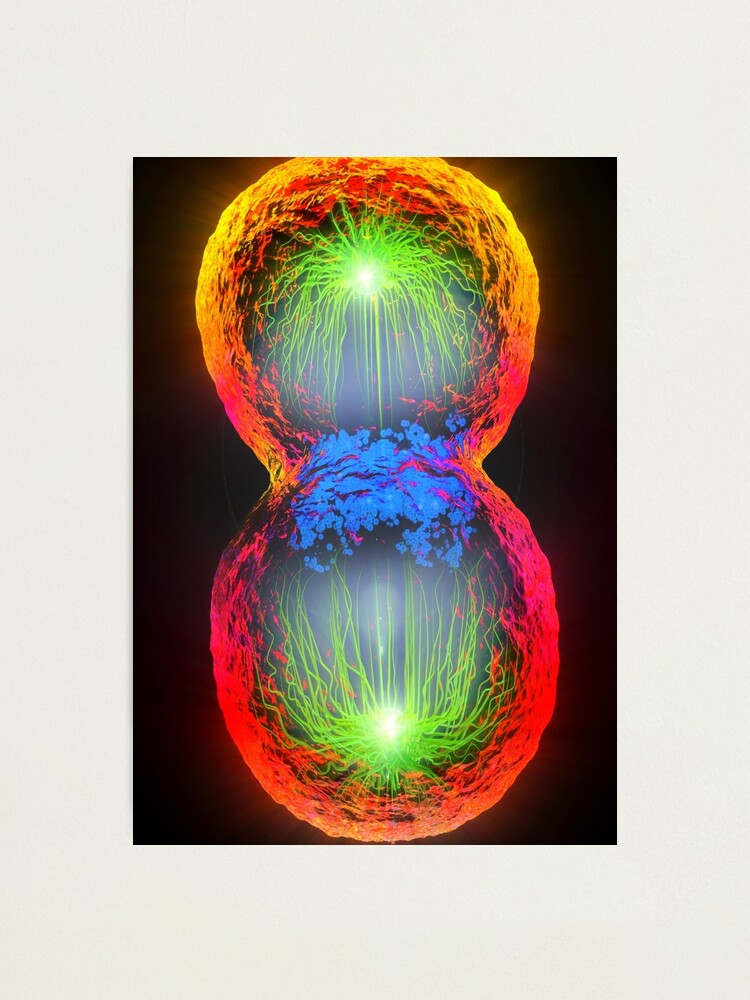The image features a vibrant and detailed depiction of cell division, presented in a canvas print with a striking contrast against a black background. Encased in a white frame adorned with a black mat, the image captures the intricate beauty of a cell in the midst of splitting. The composition is set in portrait orientation, showcasing two distinct yet connected forms resembling a figure-eight or the silhouette of cell pairs positioned one above the other.

At the core of each cell, neon green lines—resembling electric streaks—emanate from their centers, extending in opposite directions: upwards in the top cell and downwards in the bottom, representing the dynamic process of division. Where the cells meet in the center, a cloud of vivid blue light highlights the critical phase of separation.

The cells exhibit a gradient of warm colors on their outer edges, transitioning from bright red at the base to shades of orange and yellow, symbolizing the energy of the division process. The overall visual effect of the composition, combined with the layers of color and light, provides a captivating representation of biological replication suspended in a moment of transformation.